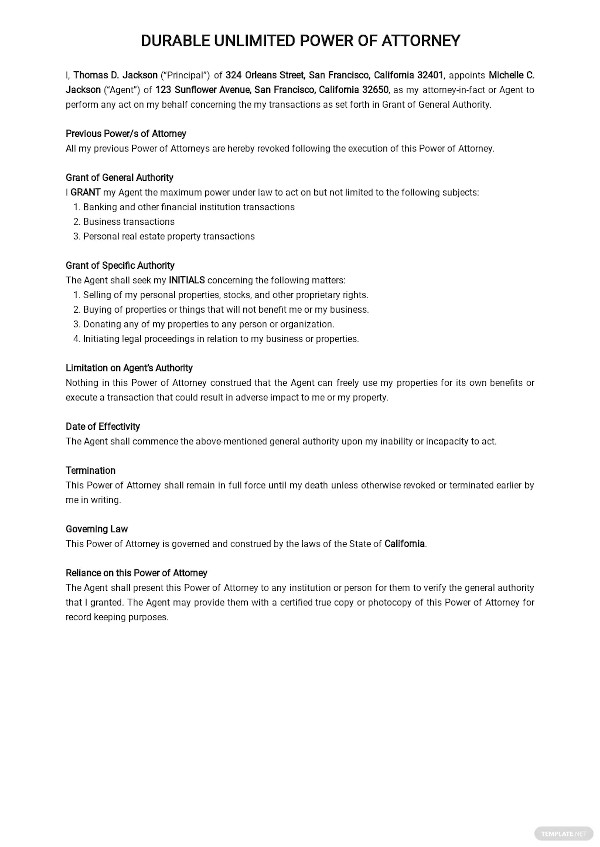A low-resolution vertical screenshot depicting a legal contract titled "Durable Unlimited Power of Attorney" against a white background. The black text details that Thomas D. Jackson, the principal residing at 324 Orleans Street, San Francisco, California 3241, appoints Michelle C. Jackson, residing at 123 Sunflower Avenue, San Francisco, California 32650, as his attorney and factor agent. The document authorizes her to act on his behalf for various transactions, specifying that all previous powers of attorney are revoked upon the execution of this new grant. The general authority granted includes the ability to perform banking and financial institution transactions, business transactions, and personal real estate property transactions. 

Specific authorities require Thomas D. Jackson's initials for actions such as selling personal property, stocks, and proprietary rights; purchasing properties that do not benefit him or his business; donating his properties to individuals or organizations; and initiating legal proceedings related to his business or properties. The document limits the agent's authority, stipulating that the agent cannot use his properties for personal benefit or engage in transactions that might adversely impact him or his properties.